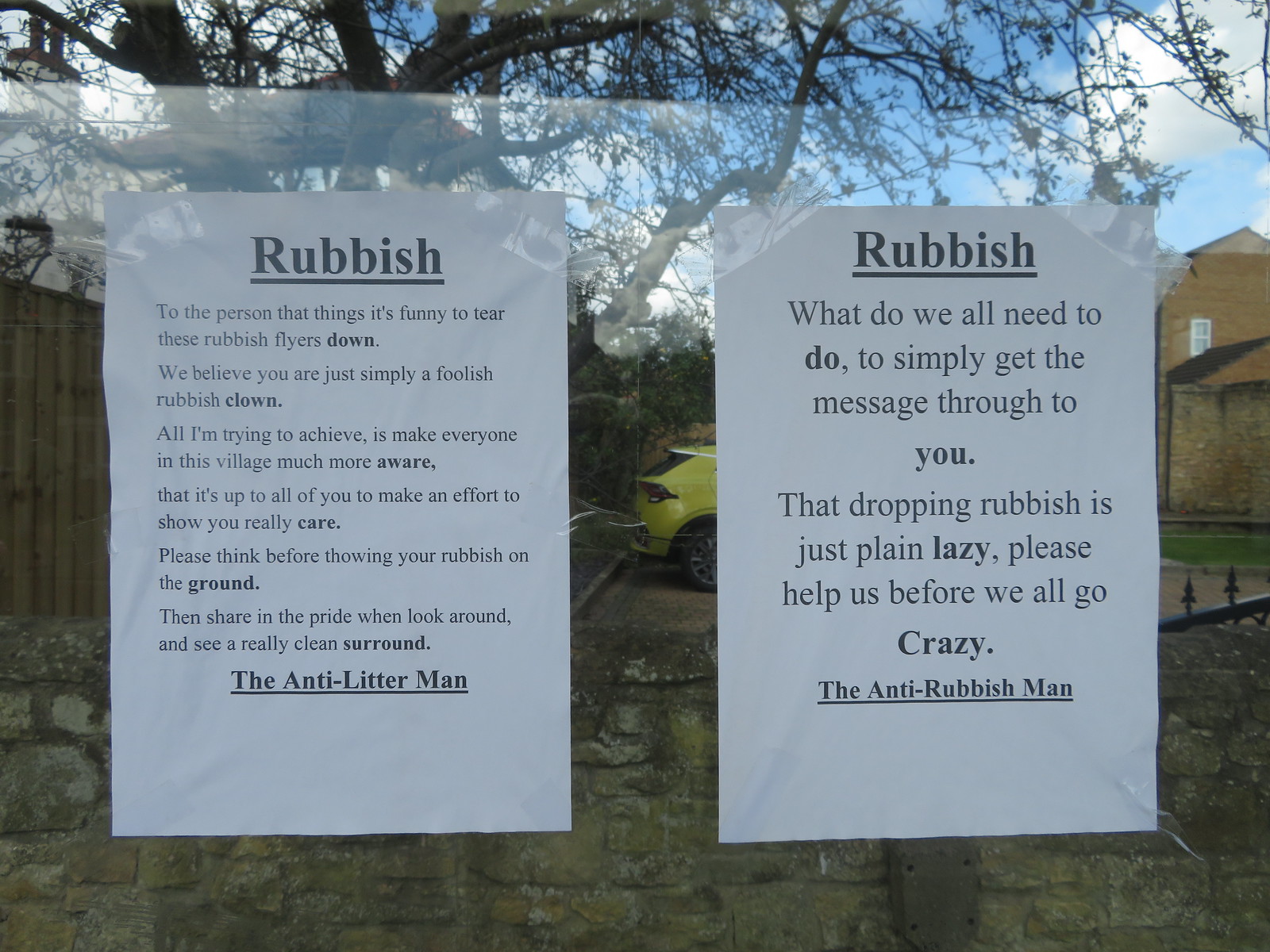In this photograph, there are two white sheets of paper with bold, black text taped to a clear glass pane. The text on each paper is underlined at the top with the word "Rubbish." The paper on the left, labeled "The Anti-Litter Man," contains a plea against littering, warning individuals against tearing down the flyers and urging the community to keep the area clean. Specific words such as "down," "clown," "aware," "care," "ground," and "surround" are highlighted in bold. The paper on the right, signed by "The Anti-Rubbish Man," echoes this sentiment, calling out the laziness of dropping rubbish and asking for help to prevent it. Key words like "do," "you," "lazy," and "crazy" are also emphasized in bold.

Visible through the glass pane is an outdoor scene featuring a partially visible yellow car, some grass and pavement, and a variety of trees. To the left and right are buildings, including one beige, possibly older structure, and some fences. The sky above is a light blue with scattered white clouds. A gray stone or brick wall, topped with protective iron arrows, frames the bottom third of the image, giving the viewer a sense of the boundary. The setting conveys a neighborhood or village atmosphere, with elements both man-made and natural contributing to the backdrop.